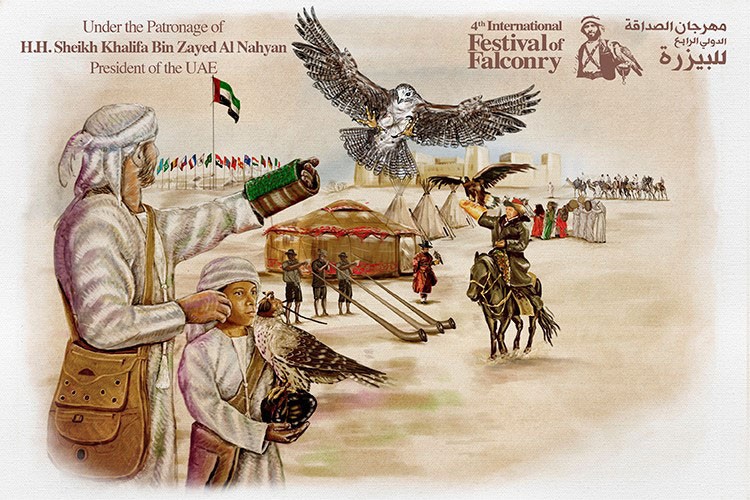The illustration depicts a scene from the Fourth International Festival of Falconry held under the patronage of H.H. Sheik Khalifa bin Zayed Al Nahyan, president of the UAE. Central to the image are an adult man and a child, both dressed in traditional Middle Eastern attire, including white headscarves and long robes. They carry large leather shoulder bags and have specialized wrist padding for falcon handling. In the center-top of the illustration, a falcon is depicted mid-flight, approaching the man's padded arm, while the boy beside him already has a falcon perched on his. The background reveals a bustling festival scene with multiple tents, a trio of men playing long horns, and another falconer on horseback, also equipped with a falcon and a glove.